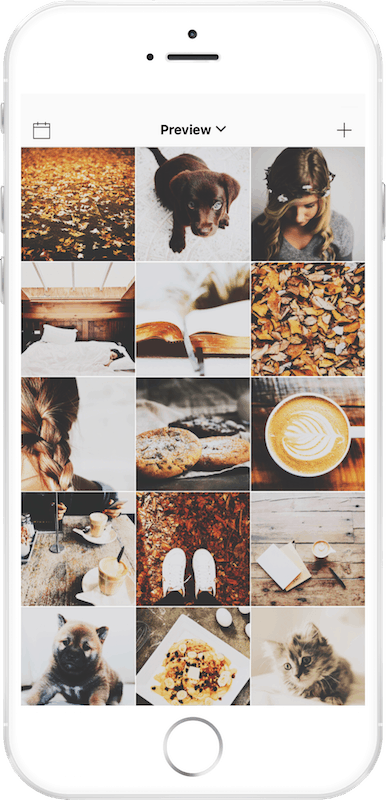The image features a white cell phone set against a plain white background. The phone has three silver buttons on its left side and one on the right. On the phone's screen, the top toolbar displays the word "Preview" centered with a downward arrow, a calendar icon to its left, and a plus button to the right.

The main part of the screen shows a colorful photo gallery comprising fifteen images, arranged in a grid of three images per row and five rows in total. The images, starting from the top left and moving right, include the following:

1. Autumn leaves scattered on the ground.
2. A small brown Labrador puppy lying on a white rug.
3. A young woman adorned with flowers in her hair.
4. A plush hotel bed in an elegantly decorated room.
5. A selection of food items elegantly arranged on white plates.
6. An adorable gray tabby kitten in the bottom right corner.
7. A small pug dog in the bottom left corner.
8. Between these two animals is a square white plate holding a dish that appears to be scallops and pasta, accompanied by a white egg in the upper left corner of the plate.

Each image is vibrant and distinct, showcasing a variety of subjects from nature and pets to culinary delights and human portraits.